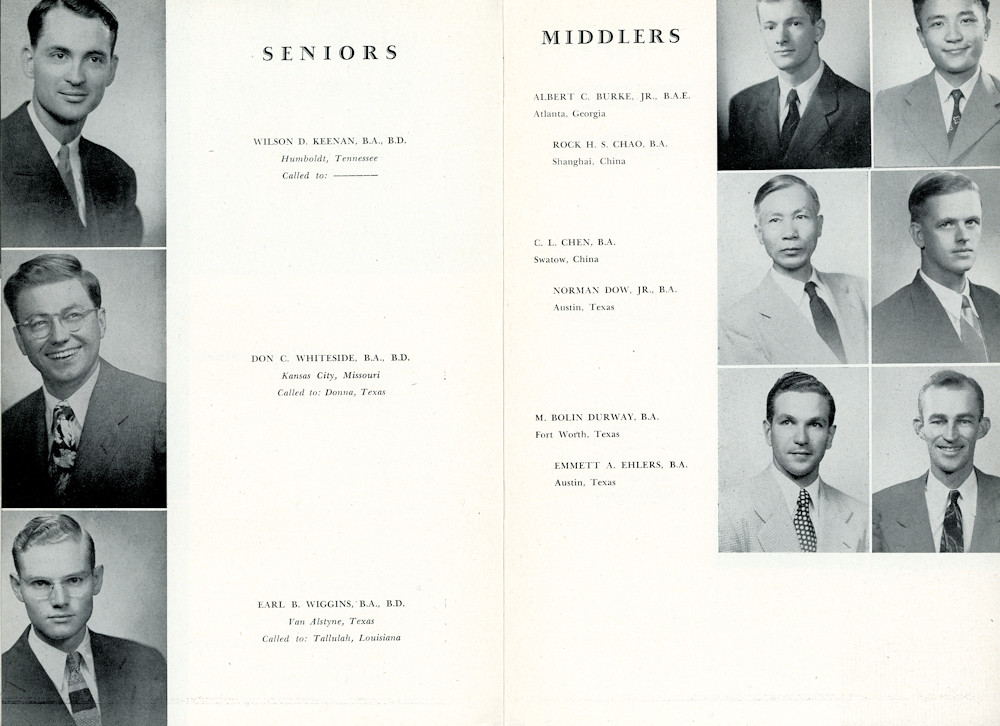This black-and-white image, extracted from an old yearbook, presents a collage of portraits divided into two categories: seniors on the left and middlers on the right. On the left side, under the heading "Seniors," we find three portraits. The first is of Wilson D. Keenan, a youthful-looking man with short, gelled-up black hair, donning a suit, identified as hailing from Humboldt, Tennessee. Next is Don C. Whiteside, an older man with glasses and a broad, toothy smile, originally from Kansas City, Missouri. The third portrait features Earl B. Wiggins, depicted with short, light-colored hair and glasses, listed from Van Alstyne, Texas.

On the right side, under the banner "Middlers," there are six photographs arranged in three rows. The top row includes Albert C. Burke, Jr., from Atlanta, Georgia, and Rock H.S. Chow from Shanghai, China. The middle row features C.L. Chen, also from China, and Norman Dow, Jr., hailing from Austin, Texas. The bottom row shows M. Bolin-Durway from Fort Worth, Texas, and Emmett A. Ehlers, likewise from Austin, Texas. All individuals in the photographs are attired in formal suits, indicative of their academic achievements and professional aspirations as noted by their accompanying degrees and locations.